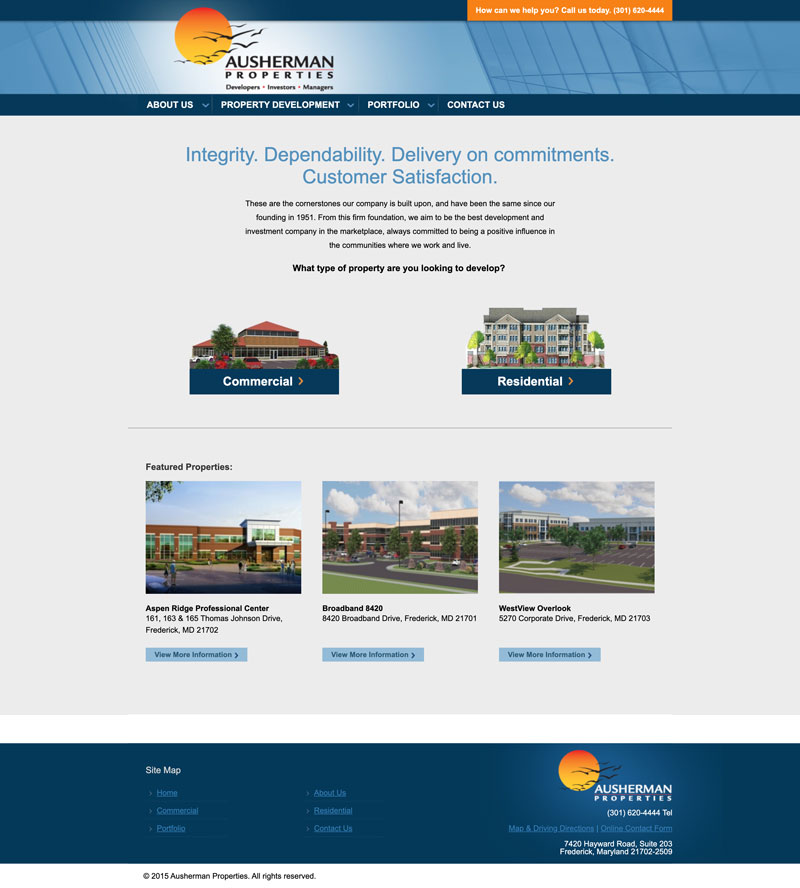The screenshot of the web page belongs to Osherman Properties, prominently featuring a vibrant design. The top section of the page is adorned with a rich blue banner that boldly poses the question, "How can we help you?" and invites viewers to call a provided phone number for assistance. Below the top banner rests another dark blue banner that addresses the company's messaging, flanked by a lighter blue banner in the center showcasing the Osherman Properties' logo. This logo includes an orange sun with birds soaring across it, reflecting the company's welcoming and aspirational brand image.

Further down, the dark blue banner at the bottom holds a navigation bar with a dropdown menu. This dropdown provides links to various sections: "About Us," "Property Development," "Portfolio," and "Contact Us," ensuring ease of access to key information.

Amidst the central white background, the company's core values are displayed prominently in blue text, highlighting "Integrity, Dependability, Delivery on Commitments, and Customer Satisfaction." Additionally, there are graphical representations for both "Residential" and "Commercial" properties. Each category is clickable, with the residential area depicted by an apartment building icon and the commercial side represented by a business building icon.

At the bottom of the web page, three featured properties are showcased: "Aspen Ridge Professional Center," "Broadband 6420," and "Westview Overlook," providing a glimpse into the diverse range of properties available through Osherman Properties.